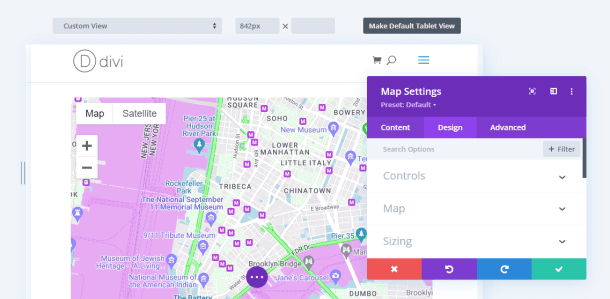This image is a screenshot of a map from an app called Divi. The app's logo, a capital "D" encircled, followed by the word "Divi" in thin, lowercase letters, is prominently displayed. The map interface is bordered in gray, reminiscent of a PDF reader's layout, enclosing the main white area where the map is displayed. The map itself is styled similarly to a standard Google Maps view, providing both road and satellite perspectives.

The depicted region appears to be New York, with identifiable landmarks such as Hudson River Park and the New Jersey transit line. Unique color coding is utilized, with the water regions shown in purple and the landmasses in gray. Roads are highlighted in white, and preferred routes are indicated in green.

Additionally, there is a pop-up overlay on the map, allowing users to modify map settings, adding to the functionality and interactivity of the application.